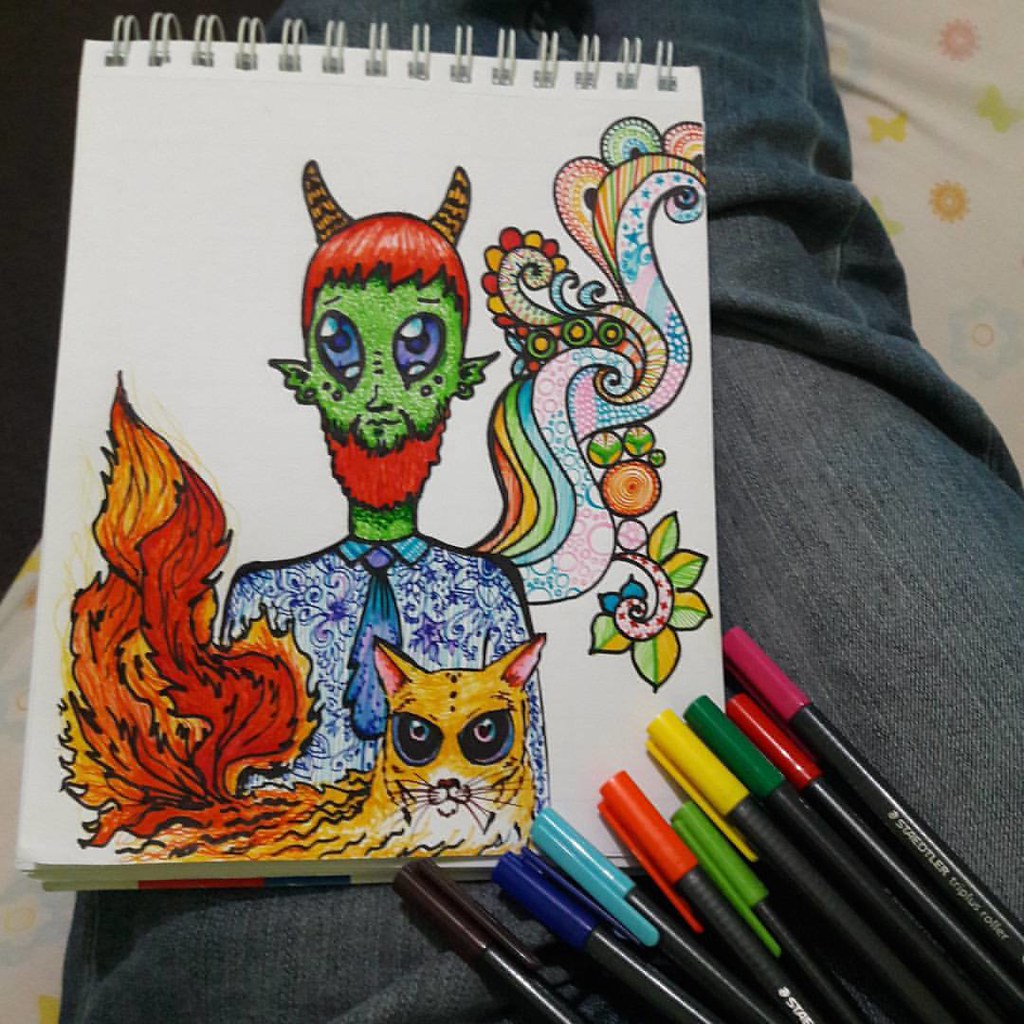In the image, a detailed drawing pad rests on someone's lap, supported by their denim-clad legs. The notebook, with white pages held together by round spiral bindings at the top, features a fantastical and psychedelic illustration. The paper captures a green-skinned alien with red-orange hair, adorned with black and orange horns and winged ears. The alien's waterdrop-like blue eyes peer out, while it dons a blue shirt with floral patterns and a purple tie. 

Below the alien, there is a fiery cat, its body seemingly engulfed in flames with a tail that blazes in red, yellow, and orange hues. The cat has darker, almost burning eyes, featuring orange fur on top and white fur with whiskers underneath, with a touch of pink inside its ears. Behind this vivid scene is a colorful, swirling rainbow in shades of orange, yellow, green, and blue, adding to the psychedelic essence of the artwork.

Surrounding the drawing, and scattered on the lap of the artist, are an array of colorful markers, including purple, red, green, yellow, light green, orange, light blue, dark blue, black, brown, teal, and burgundy. The artist appears to be seated on a bed adorned with a white comforter that has multicolored patterns featuring yellow suns, butterflies, and blue flowers, adding a homey touch to the creative setup.